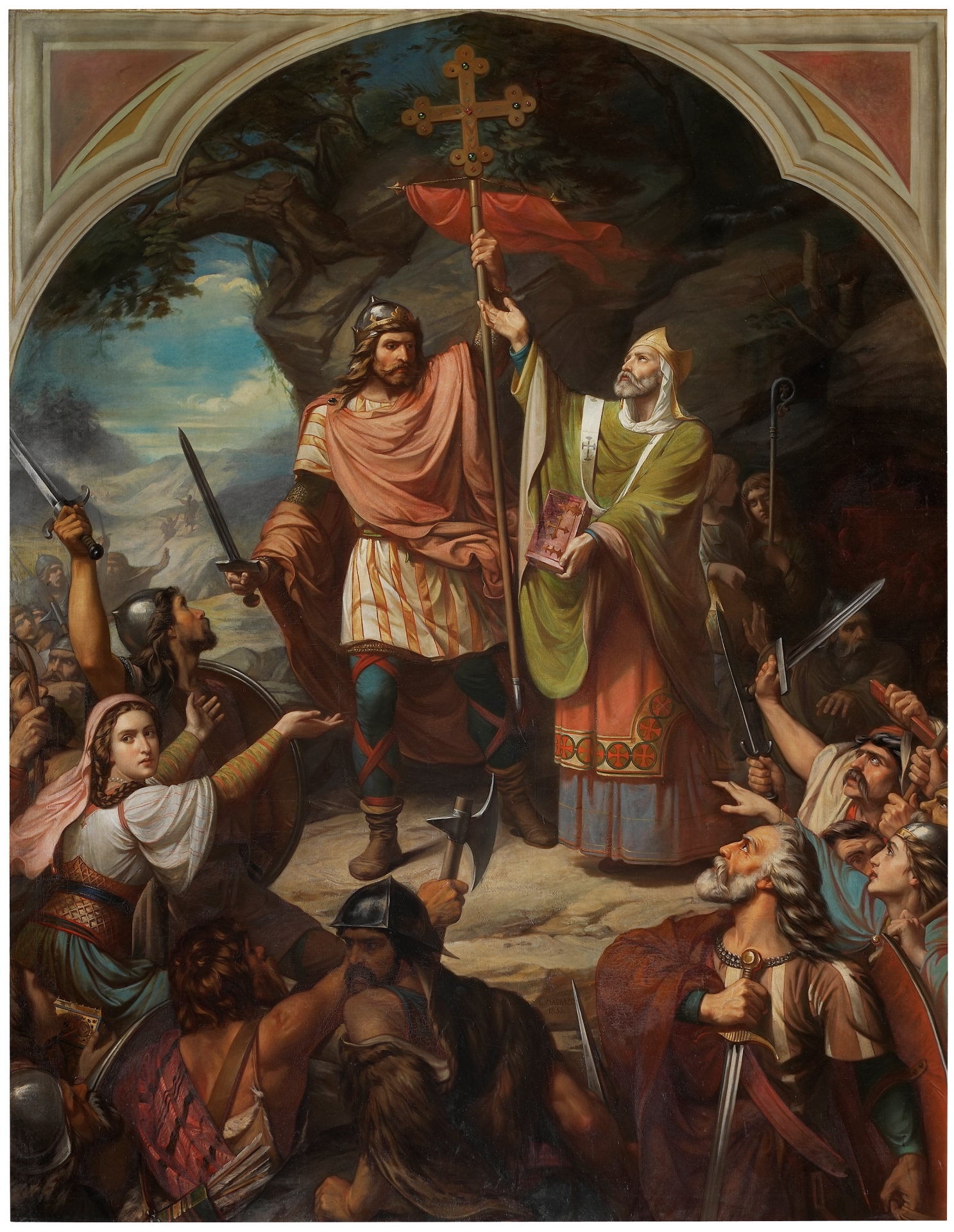This detailed painting, inset within an arch-like cornice at the top corners, depicts a dramatic historical scene. Center stage, on a rocky ledge with a sheer cliff backdrop, stand two prominent male figures. The man on the left is a warrior, identifiable by his metal helmet, teal leggings, and brown boots. His outfit includes a white and gold striped tunic skirt and a red shawl draped over his chest. In his right hand, he brandishes a sword, while his left hand holds a staff capped with a cross. To his right stands a religious leader, dressed in green robes and adorned with a gold crown. This figure holds a book in his left hand and raises his other hand towards the cross atop the staff shared with the warrior.

Below the ledge, a crowd gathers, composed of men and at least one woman. These figures are armed with various weapons—swords, axes, knives—and wear helmets, their expressions a mix of anger and urgency. One man prominently points a battle axe at the priestly figure, while a woman on the left stretches her arms out towards the central men. The vivid colors and intricate details of the painting highlight the tension and energy of the scene, capturing a moment rich with historical and dramatic significance.